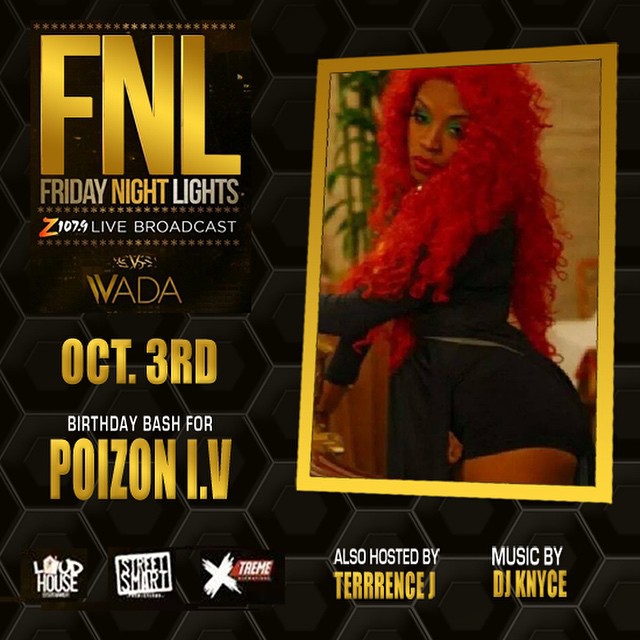The poster is designed to promote an electrifying club event. The background features a dark honeycomb structure, with hexagon patterns creating a modern and edgy feel. On the right side, set within a bold yellow frame, is a picture of a woman with striking bright red hair. 

The event details are prominently displayed. It is hosted by Terrence J with music by DJ K-Nyce. The left side of the poster announces that this is an FNL (Friday Night Lights) live broadcast event. The date, October 3rd, is highlighted in vivid yellow for easy visibility. This special occasion is a birthday bash for Poison Ivy, spelled uniquely as P-O-I-Z-N I.V., who is likely the woman featured in the image. 

Overall, the poster conveys an exciting and vibrant atmosphere, promising an unforgettable night.